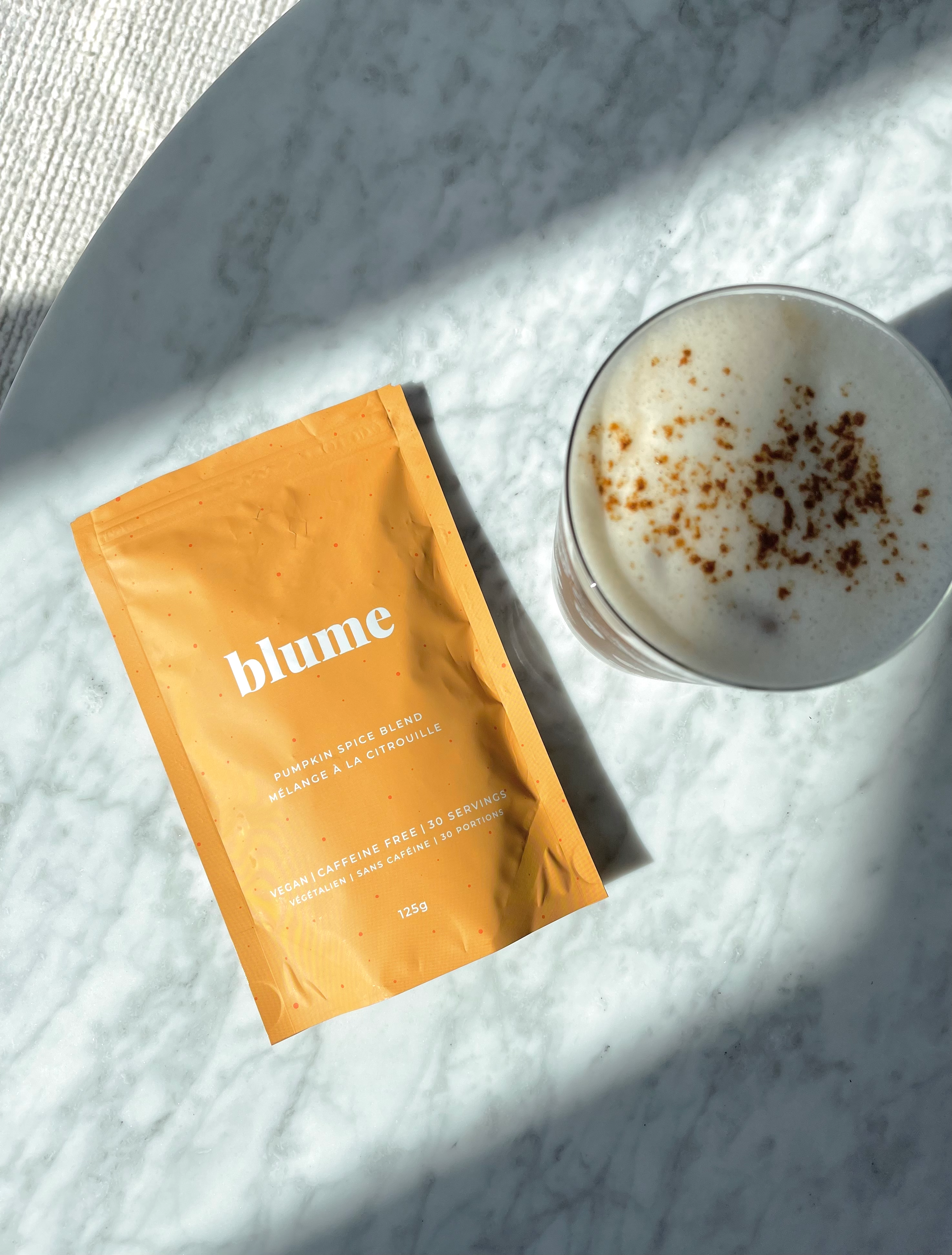The image showcases an artistic arrangement featuring an orange package labeled "Bloom" alongside a drink topped with a contrasting layer of white foam and a sprinkle of cinnamon or a similar powder. Set on a marbled table with a rug in the background, the vibrant package serves as the focal point. It details "Pumpkin Spice Blend" and "Melange a la Citrouille," noting that it is vegan, caffeine-free, suitable for vegetarians, and contains 30 servings, weighing 125 grams. The drink, likely enhanced by the spice blend, appears untouched and is filled to the brim. The clean white foam on the drink stands out against the darker powder, enhancing the visual appeal of the scene.